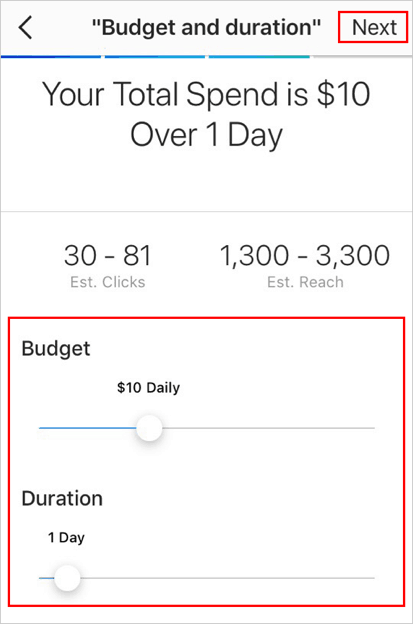The image displays a budgeting and duration interface. In the upper left corner, there is a back arrow button, followed by a top bar that reads "Budget and Duration" in black font, with 'Budget' having a capital B. Adjacent to this on the top bar is a "Next" button, highlighted with a red outline around it, featuring a capital N in black font. 

Below the top bar are four horizontal lines, the first three from the left are colored blue. Underneath these lines, there is a text block that states, "Your total spend is $10 over one day," written in black font. 

A light gray separator bar follows, displaying "30 to 81 estimated clicks." Below this bar is a budget slider outlined in red, set to $10 daily. Directly underneath the budget slider is another slider for duration, set to one day.